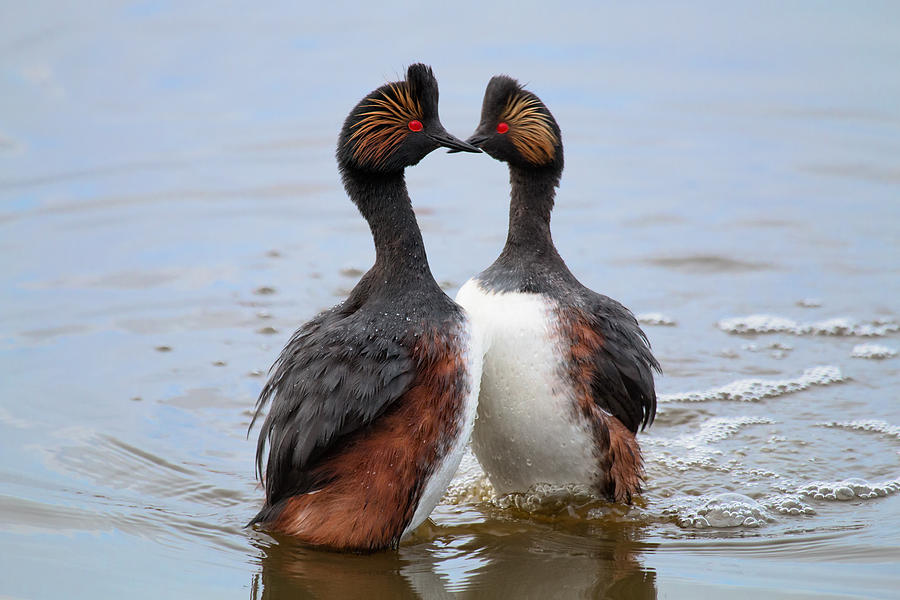This is a detailed close-up photo of two crested ducks engaged in a mating dance in the water, appearing to kiss with their beaks touching and chests pressed together. Both ducks have distinctive black heads, necks, and wings, contrasted with auburn feathers on their bodies and white chests and stomachs. The most striking feature is the flamboyant gold spiky feathers fanned out around their deep red eyes. The water they're standing in is brown and murky, with visible ripples and bubbles, reflecting the light from above. The ducks' identical coloration and synchronized posture create a captivating symmetry, making the image both elegant and intimate.